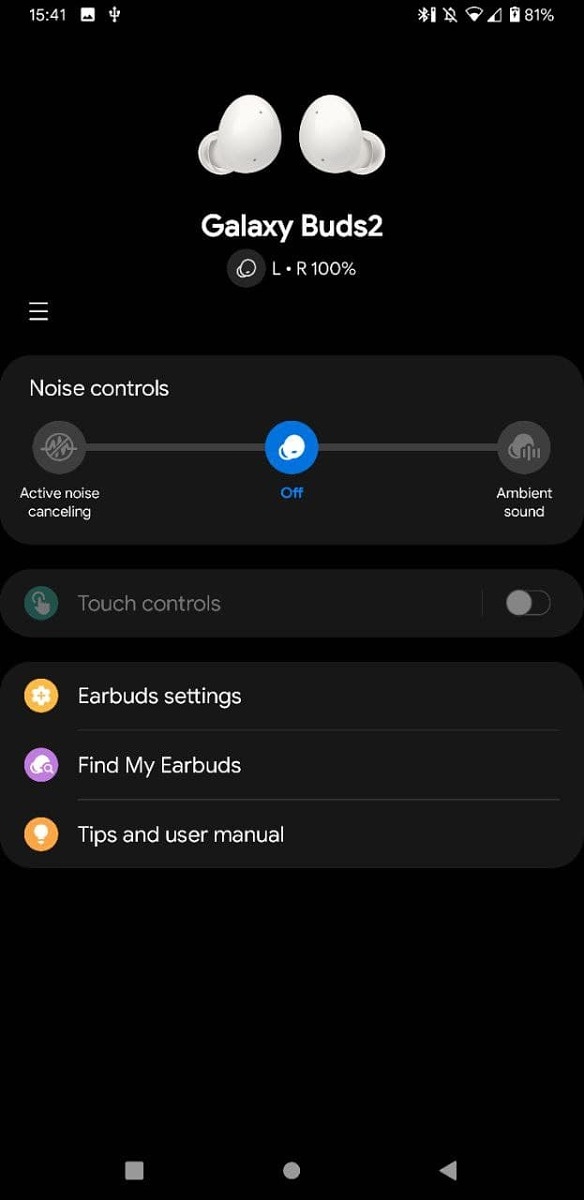The image is a screenshot taken from an iPhone, displaying the battery life at 81%, with a strong network connection. The time is shown in military format as 15:41. The main subject of the image, set against a black background, is the interface for Galaxy Buds 2. At the top, there's an illustration of two earbuds labeled "Galaxy Buds 2," each indicating a 100% charge for both the left and right bud. Below this, there are three control options within a section titled "Noise Controls." The first option, "Active Noise Canceling," has a gray button. The second option, "Off," is highlighted with a blue button and includes an image of the Galaxy Bud. The third option, "Ambient Sound," also features a gray button along with a grayscale image of a Galaxy Bud.

Further down, there's a section named "Touch Controls," which is turned off and marked with a green insignia. The next section, "Earbud Settings," is represented by an orange icon with a star in the middle. "Find My Earbuds" features a purple icon with a white image. Finally, there's a "Tips and User Manual" section, symbolized by an orange circle with a white element in the middle.